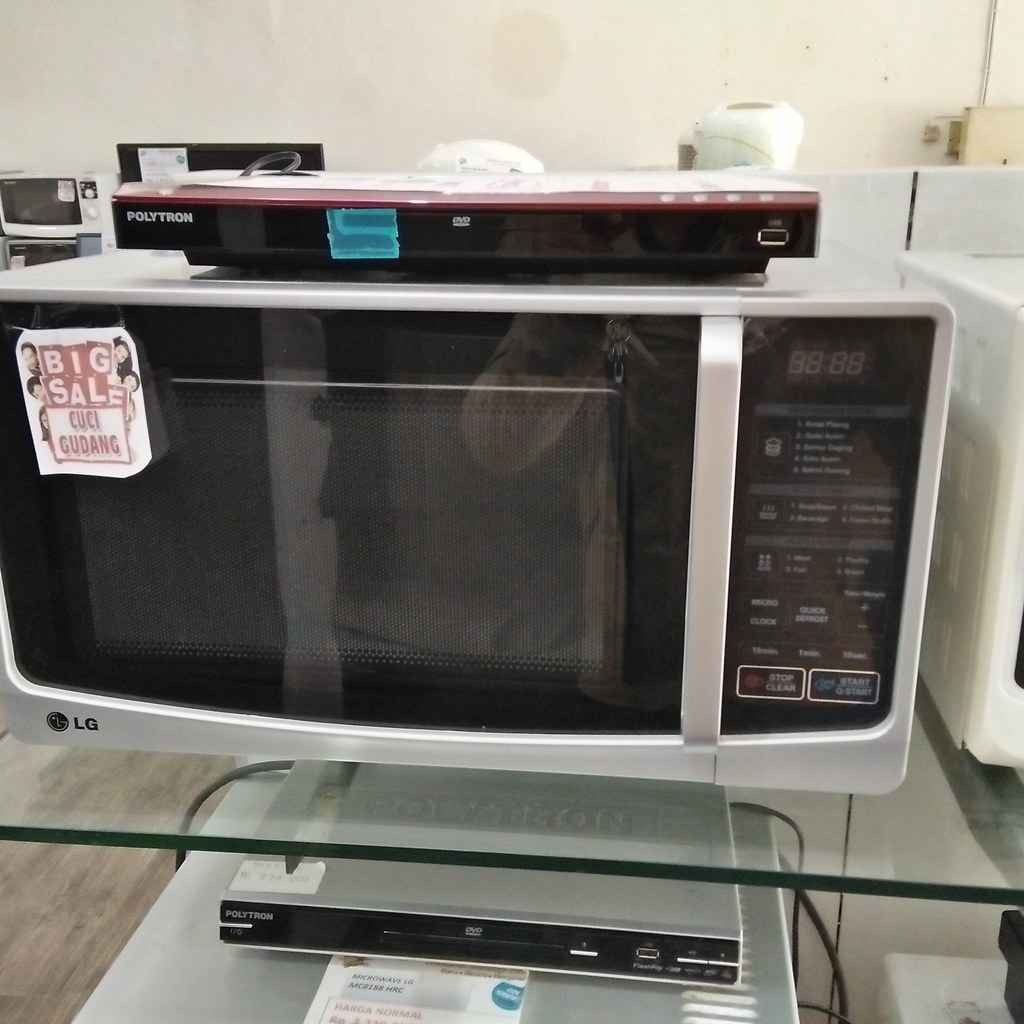The image captures a detailed scene within an appliance store. At the forefront, there is a white LG microwave with a black door and control panel, positioned on a glass display shelf. Placed atop this microwave is a Polytron DVD player, and beneath the shelf sits another slightly different Polytron DVD player. Attached to the left side of the microwave is a label that reads "Big Sale" with the words "CUCI" and "GUDANG" below it, and three heads appearing from the side of the label. Surrounding the main microwave are various other small kitchen appliances, including rice cookers and other microwaves, indicating the store's specialization in kitchen appliances. The backdrop of the scene features additional microwaves and potential air fryers, all set upon a floor with a fake wood pattern and against a white wall. The environment clearly showcases the products in a neatly organized manner, typical of an appliance retail setting.